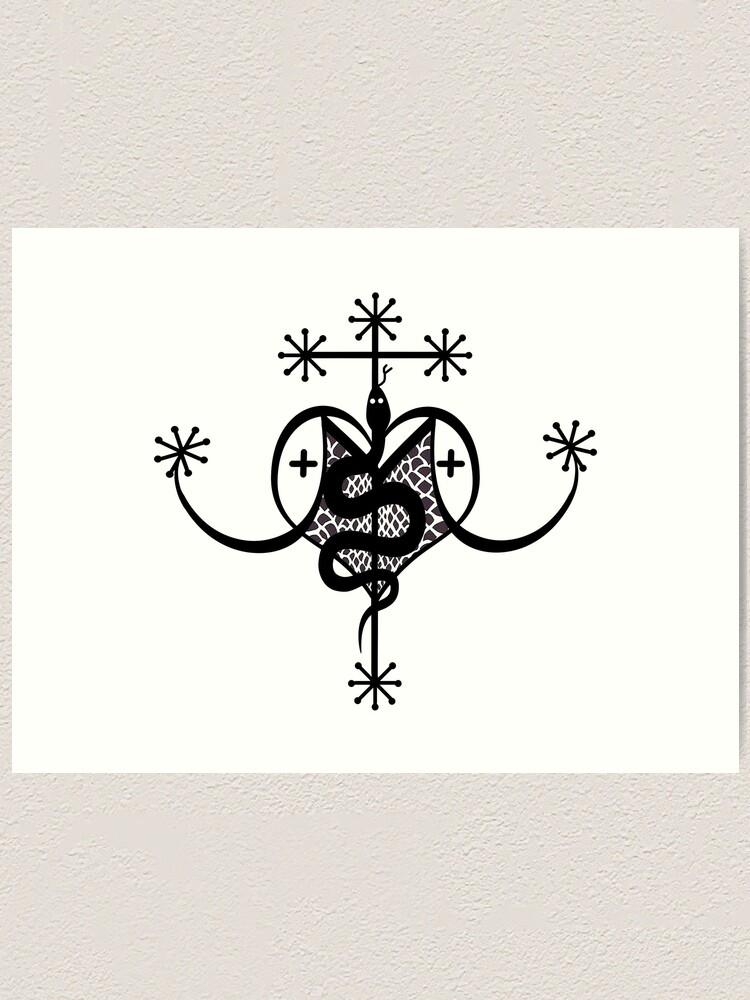This detailed black and white graphic, rendered on a standard white piece of printer paper, is displayed on an off-white plaster wall, revealing some of the wall’s texture. At the center of the graphic is a heart, filled with a pattern reminiscent of snake scales and dotted with two small black crosses. A central cross extends vertically through the heart, ending in radial, star-like elements with rounded edges, marked by black lines and dotted tips. Adding to the complexity, a black, serpentine figure undulates through the heart and cross, mimicking the motion of a sidewinder snake. Flanking the heart's sides are two looping curves. The entire composition is framed against the textured plaster wall, contributing to its stark and ritualistic visual impact.